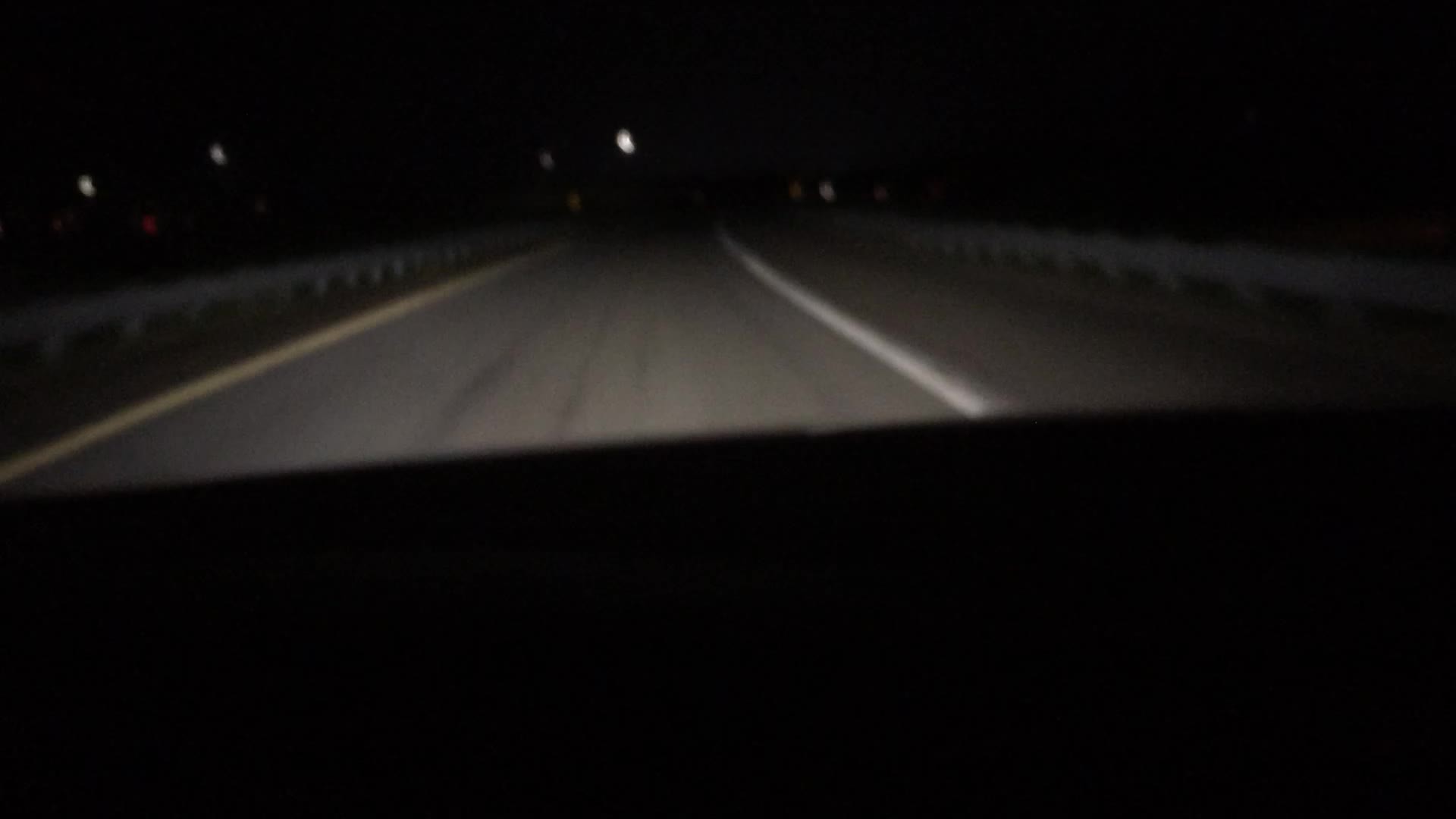The photograph, taken at night from inside a car, prominently features the vehicle's dashboard at the bottom, occupying nearly half the image. The picture looks down a single-lane gray road illuminated by headlights, revealing solid white lines on both sides. On either side of the road, there are small metal fences or gray-colored guardrails, with a hint of grass and possibly a yellow curb on the left. The background is pitch black, punctuated by various dots of light: a bright white dot in the distant center, flanked by two smaller white dots and a red dot towards the upper left. Additional lights are also visible near the top right and center left of the image. The asphalt displays some dark streaks, enriching the scene with realistic road texture.